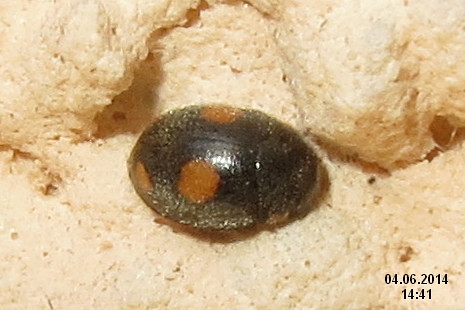The image features a reverse ladybug-like black beetle resting on a light cream, almost beige, stone formation with a bumpy texture, resembling a porous yellowish marshmallow. The beetle, oval in shape and divided into multiple sections separated by fine lines, displays distinctive markings: an orange dot on the top, bottom, and back, with additional yellow specks scattered across its body. A small white light reflection is visible at the center of the beetle. Nestled in a slight cavity within the stone, the insect is near a narrower hole on the right side of the formation. The photograph is timestamped at the bottom right corner with the date 04.06.2014 and the time 14:41.